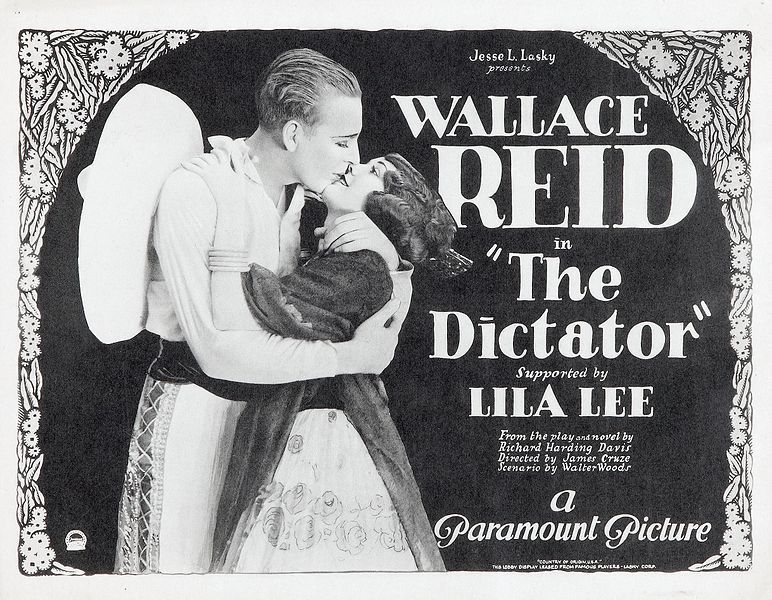This black-and-white landscape-oriented poster is a vintage advertisement for the film "The Dictator," starring Wallace Reid and Lila Lee. The poster, likely from the 1920s, features intricate flowery borders along the left and right sides, and a bit more on the top. In white text at the top, it reads "Jesse L. Lasky presents," followed by "Wallace Reid in 'The Dictator'" in large letters. Below, it states "Supported by Lila Lee," and provides additional credits: "From the play and novel by Richard Harding Davis," "Directed by James Cruze," "Scenario by Walter Woods," and "A Paramount Picture," all in a smaller white font.

The central image shows a romantic scene: a couple kissing, with the man on the left holding the woman with his right arm around her back. The man is dressed in a white long-sleeve shirt and white pants, with a sombrero tied to his back, evoking a Mexican aesthetic. The woman wears a flower-patterned dress with a darker-colored shawl over her shoulders, and her short hair is styled in curls around her face. The background of the poster is black, highlighting the white font and intricate floral designs on the borders, enhancing the vintage, romantic ambiance of the poster.